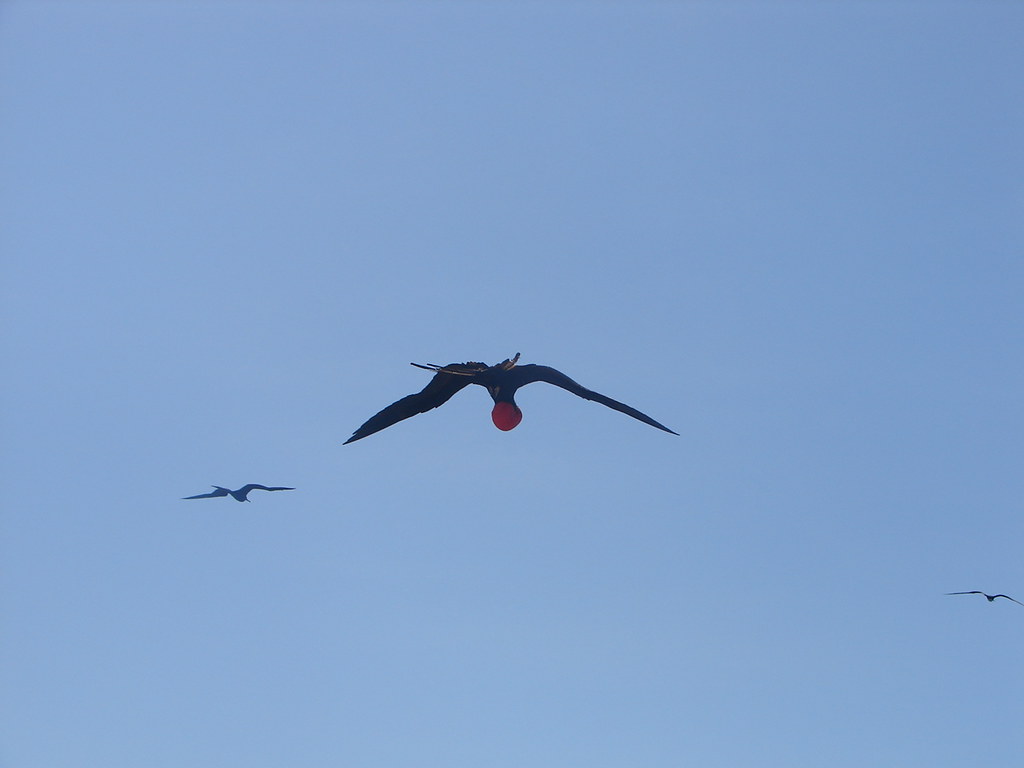In this striking image, three birds soar against a bright, cloudless blue sky. The focal point of the scene is a prominent seagull in the center, with long, dark wings and an elongated beak. This bird is gripping a round, red object in its talons, which adds a splash of color to the composition. To the left of the central bird is a smaller seagull, appearing distant as it flies away. Another seagull, also small and in the distance, is positioned in the bottom right corner, further emphasizing the vast, open expanse of the sky. The overall scene is serene and detailed, with the contrast of dark birds against the vibrant blue sky creating a visually engaging photograph.